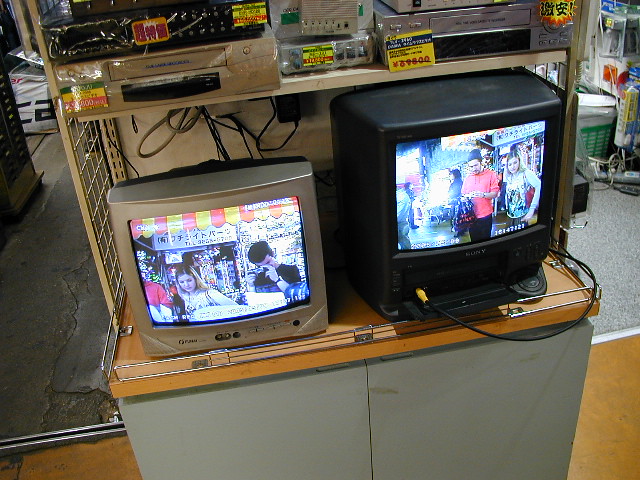The photograph captures an indoor scene of a cluttered store or a bargain resale shop. Central to the image is a tan, metal shelf positioned on top of a grayish cabinet with two white doors and a fake wood top bordered by metal. The cabinet rests on a tan linoleum floor. Displayed prominently on the shelf are two old tube televisions; the smaller, silver TV stands on the left, while the larger black TV is on the right. Both sets are on, depicting colorful street scenes with people shopping, possibly resembling security camera footage.

Above the televisions are several VCRs from the early 90s, some in saran wrap, each with yellow price tags indicating that they are for sale. Cords from the TVs and VCRs dangle in front, suggesting connections to external devices like DVD players. The background reveals a cluttered store environment, slightly out of focus, with sections of cracked wood flooring to the left and gray carpeting to the right. Yellow price tags with crossed-out prices further suggest this setup is part of a resale section, emphasizing the older technology's affordability.